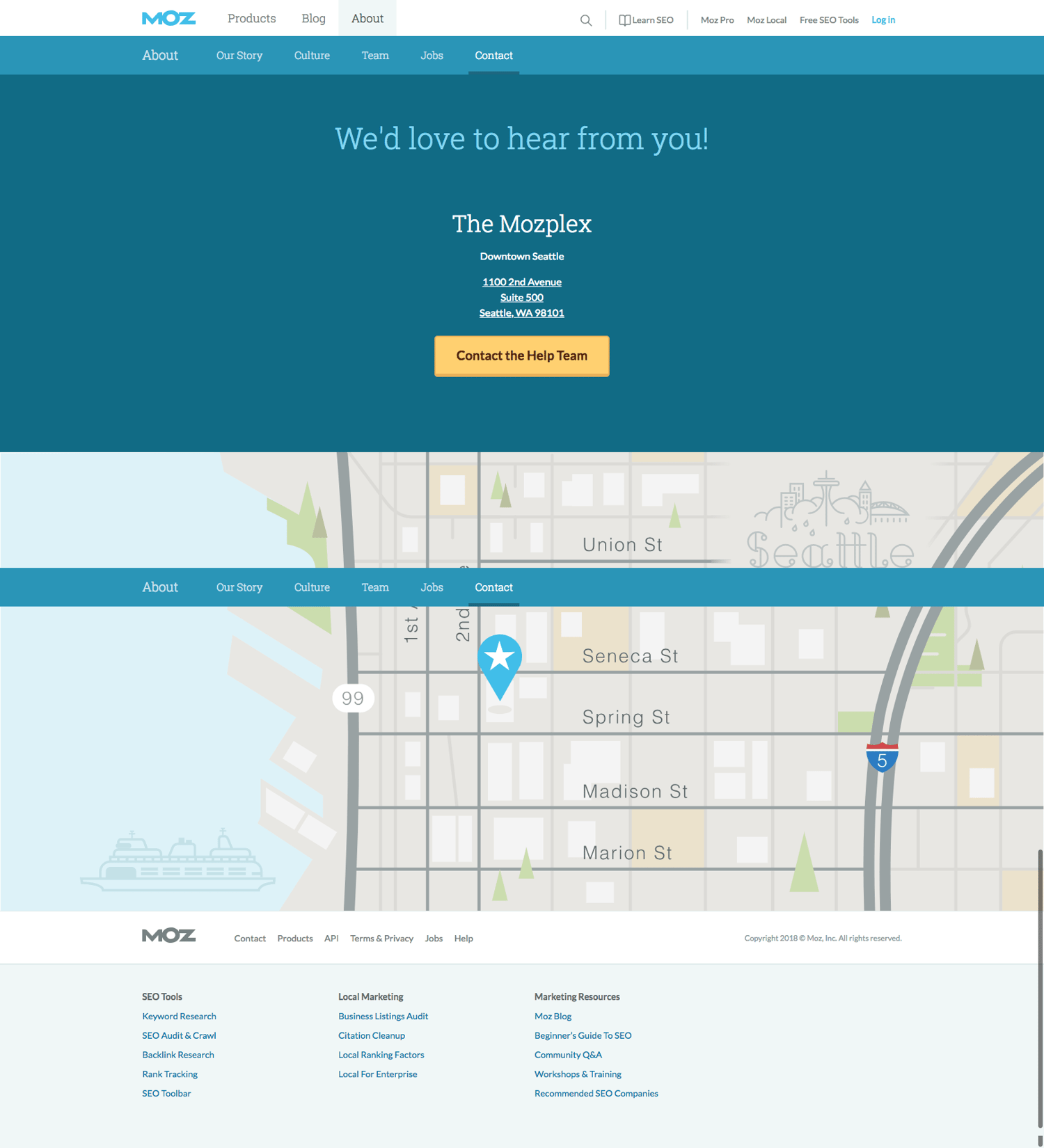This image is a detailed screenshot of a web page from the Moz website. At the top left corner, the word "MOZ" is prominently displayed in blue. Spanning the top of the page from left to right are navigation links labeled as "Products," "Blog," and "About," followed by a search bar. Adjacent to the search bar are additional links: "Learn," "SEO," "Moz Pro," "Moz Local," and "Free SEO Tools." A blue "Login" button is positioned at the far right of this navigation strip.

Directly beneath this, there is a light blue stripe containing another set of links labeled "About," "Our Story," "Culture," "Teams," "Jobs," and "Contact," with "Contact" specifically highlighted. Below this stripe, a message reads, "We'd love to hear from you," followed by the address for the Mozplex in downtown Seattle. Next to the address is a yellow button labeled "Contact the Help Team."

An image of a map with a pinpoint indicating Moz's location in Seattle is displayed under the text. There is another navigation stripe overlaid on the map, bearing the same links: "About," "Our Story," "Culture," "Team," "Jobs," and "Contact." At the very bottom of the page are various company links, including "Marketing Resources," "Local Marketing," and "SEO Tools," all in very small blue hyperlinks, making them difficult to read.

Additionally, the map features a whimsical portrayal of a cruise ship drawn in the ocean area off the coast of Seattle.